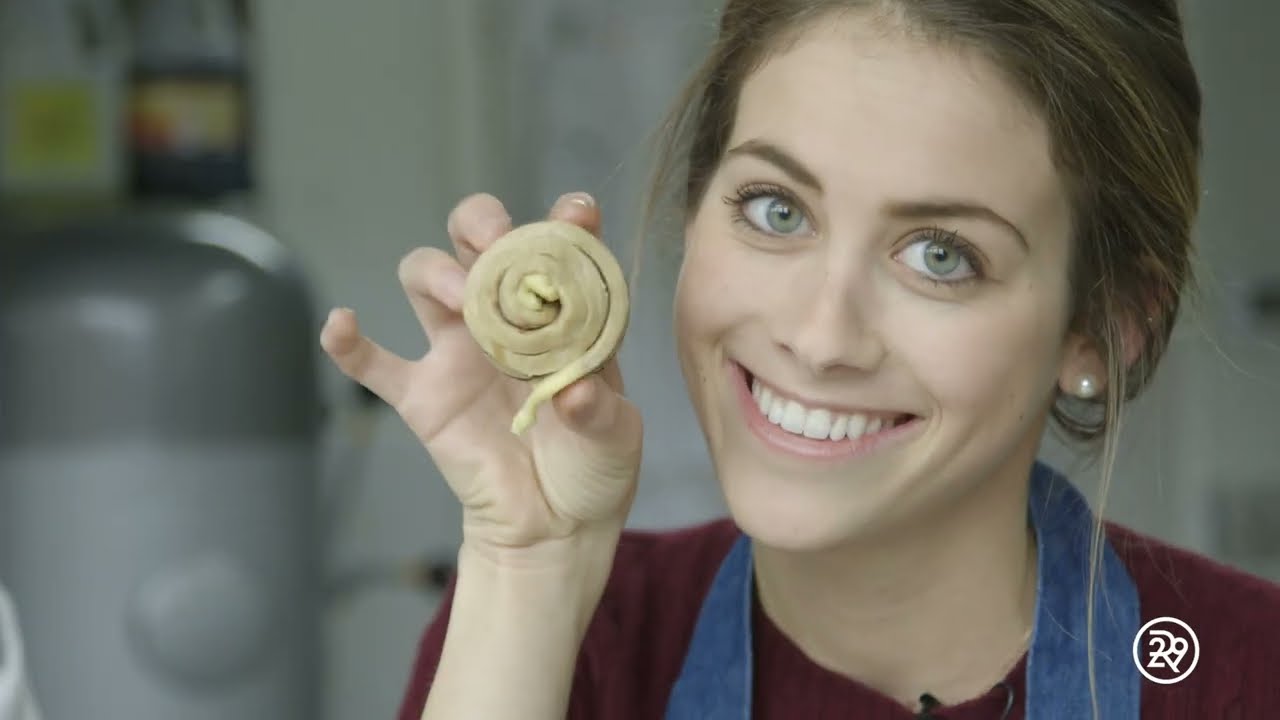The image is a close-up of a young woman in her late 20s, occupying most of the right-hand side of the picture. She has brown hair with lighter highlights, pulled up into a bun, and blue-green eyes. Her makeup includes white teeth and pink lips, complemented by a pearl earring visible on one ear. She is smiling warmly at the camera, showcasing her flesh-colored lipstick. She is dressed in a denim apron over a maroon or cranberry long-sleeve shirt. The apron covers her shoulders and neck.

The woman holds an unbaked cinnamon roll in her right hand, with the dough rolled into a circular, snail-like shape. Her arm is raised, prominently displaying the cinnamon roll in front of her. Behind her, there is a blurry background that seems to be a large commercial kitchen with white and silver walls and a silver machine with a black handle.

In the bottom right corner, there is a circular logo featuring a fancy font that resembles "2R9" or "U29," possibly hinting at some sort of branding or advertisement, likely for a cooking show or bakery shop. The overall setting and her attire suggest she is engaged in a culinary activity.